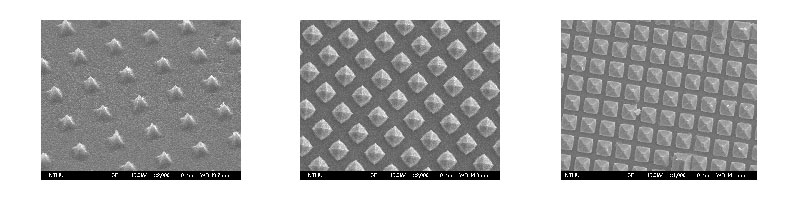The image comprises three textured panels displayed against a plain white background, forming a horizontal sequence with white spaces separating them. Each panel measures slightly over an inch in width and height, with a thin black footer at the bottom containing small, illegible white text. All panels feature intricate geometric textures on a light to medium gray background.

The leftmost panel depicts an isometric view of equilateral pyramid-like protrusions arranged in neat rows, resembling pointed mountaintops or frilly, bush-like shapes spaced relatively far apart. The middle panel offers a more detailed top-down perspective of similar pyramid formations, highlighting the square bases with tips pointing upwards, in a denser, grid-like arrangement. The rightmost panel also presents a top-down view but from a higher vantage point, revealing a larger, tighter grid pattern with numerous closely-packed pyramidal shapes divided by thin gray lines. The composite image provides a fascinating study of texture and perspective, showcasing the progression of spatial density and viewpoint in geometric formations.